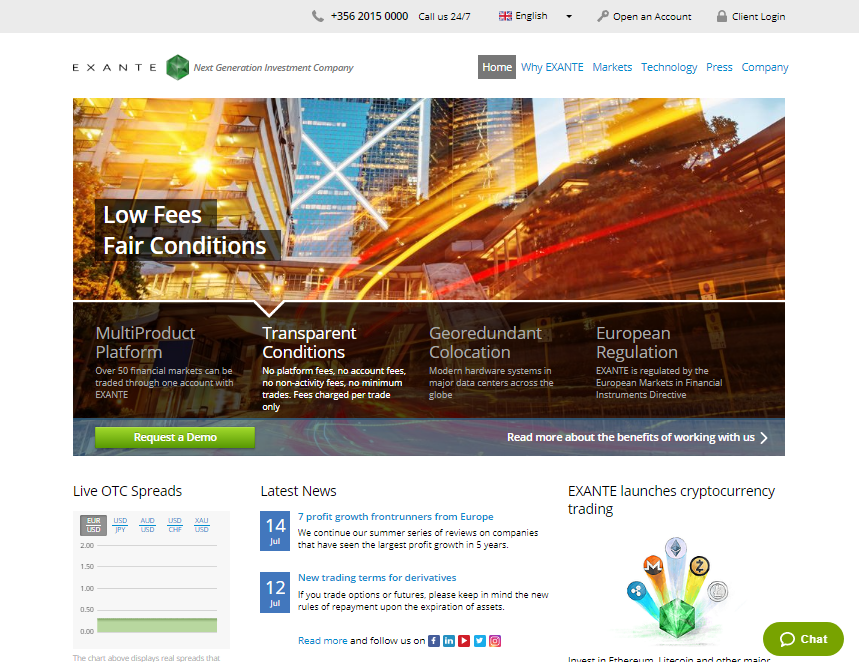Screenshot of Exante Website - Next Generation Investment Company

The image showcases a screenshot of Exante's official website, an investment company positioned as "Next Generation." The top bar of the website is light gray, featuring a prominent emerald hexagon logo next to the company name "Exante." 

The top bar displays a phone number, "+356-2015-000," available for calls 24/7. It includes a context menu adorned with an English flag signifying language options, an "Open an Account" button featuring a key icon, and a "Client Login" button with a block icon.

The primary navigation menu sits below the top bar, with the "Home" tab currently selected, highlighted in white lettering against a gray background. The subsequent tabs, written in blue and listed from left to right, include "Why Exante," "Markets," "Technology," "Press," and "Company."

The main visual of the page is a vibrant cityscape with streaking lights, symbolizing rapid movement and progress. Below this image, a black box with white lettering touts "Low fees, fair conditions." Additional text in light gray or white elaborates on Exante's offerings: a multiproduct platform providing access to over 50 financial markets, transparent conditions, no platform or account fees, no private activities, and no minimum trades, with fees charged per trade only.

Further details include mentions of "Modern Harvard, Simpsons, and major data centers across the globe," and that Exante operates under "European regulation," being overseen by a European markets financial institution directive.

A green box invites users to "Request a demo" and "Read more about benefits working with us." Below this section, there is a live OTC spread display and a "Latest News" widget, with an announcement about Exante launching cryptocurrency trading. A chat option appears in the bottom right-hand corner, represented by a green bubble containing a white speech bubble icon.